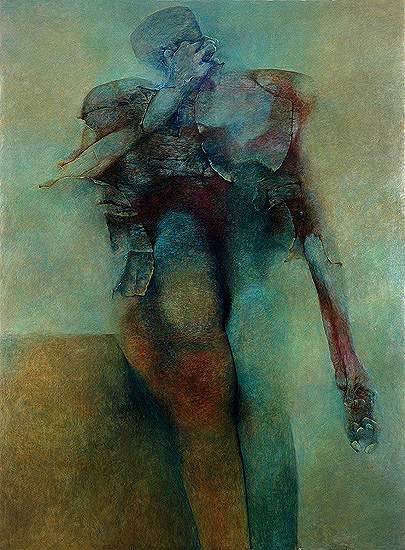In this surreal and abstract painting, a human-like figure dominates the scene, positioned upright and leaning against a rectangular object at the bottom left corner of the canvas. The figure, characterized by a bald head, displays a distressed or contemplative expression as its right hand rubs its eyes while the left hand, skeletal and elongated, hangs by its side, holding an indistinct object. The upper torso and shoulders exhibit a patchwork or cracked appearance, seemingly made of different materials, giving it a stone-like texture. The legs are unnaturally long and thick, merging directly into the chest without a visible crotch region, emphasizing a distorted human form. The overall color palette of the painting is muted, predominantly featuring shades of orange, blue, green, and brown, with the background blending greens, yellows, and blues. The depiction of the body parts is skeletal in some areas, particularly the hands and head, while the head itself is unusually flat, tilted to one side, and detailed with multicolored, cracked impressions.